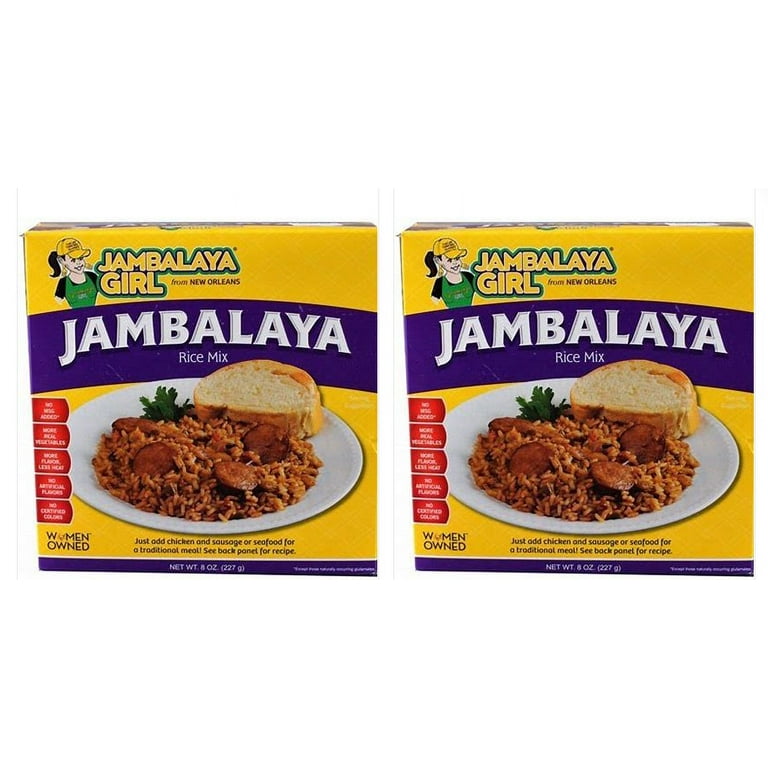The image showcases two identical boxes of Jambalaya Rice Mix from the brand Jambalaya Girl, positioned side by side against a white background. Each box features a prominent text at the top left corner stating "Jambalaya Girl from New Orleans," accompanied by a cartoon image of a woman wearing a yellow baseball cap, a black shirt, and a green apron with a ponytail. Below this, the product name "Jambalaya Rice Mix" is written in white text on a purple banner. The center of the box displays a photograph of jambalaya rice with sausage slices and green herbs, served on a white plate alongside a thick slice of oval-shaped white toast. The bottom left corner of each box includes the claim "Women Owned," emphasizing the company's ownership. The packaging is predominantly yellow with accents of blue, purple, red, and green, with some red tabs on the lower left providing additional health claims, though the text is not legible.